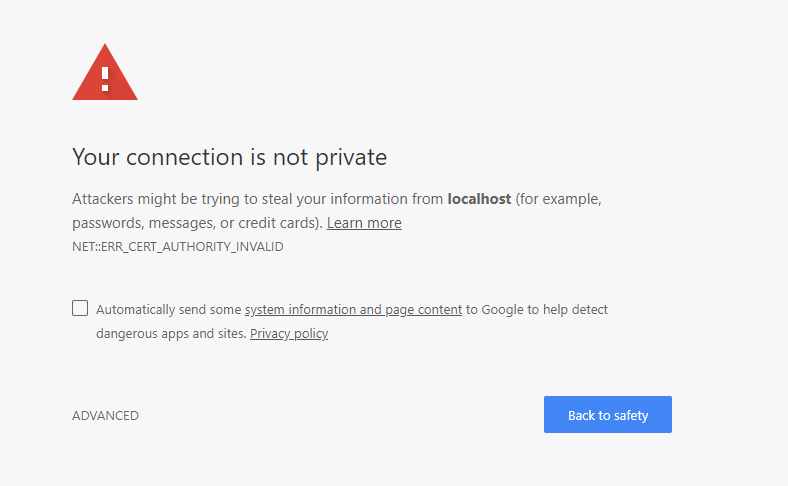A screenshot displaying a browser warning message, indicating a potential security issue when attempting to access a website. The top left corner features a prominent red triangle with an exclamation point. Below, bold text states "Your connection is not private." The message warns, "Attackers might be trying to steal your information from localhost, for example, passwords, messages, or credit cards," followed by a link to "Learn more." Further down, the error code "NET::ERR_CERT_AUTHORITY_INVALID" is displayed. A checkbox option, currently unselected, offers to "Automatically send some system information and page content to Google to help detect dangerous apps and sites," accompanied by a "Privacy Policy" link. At the bottom, two interactive buttons are available: "Advanced" on the left, which provides an option to proceed to the site despite the warning, and "Back to safety" on the right, which redirects the user back to the previous page.